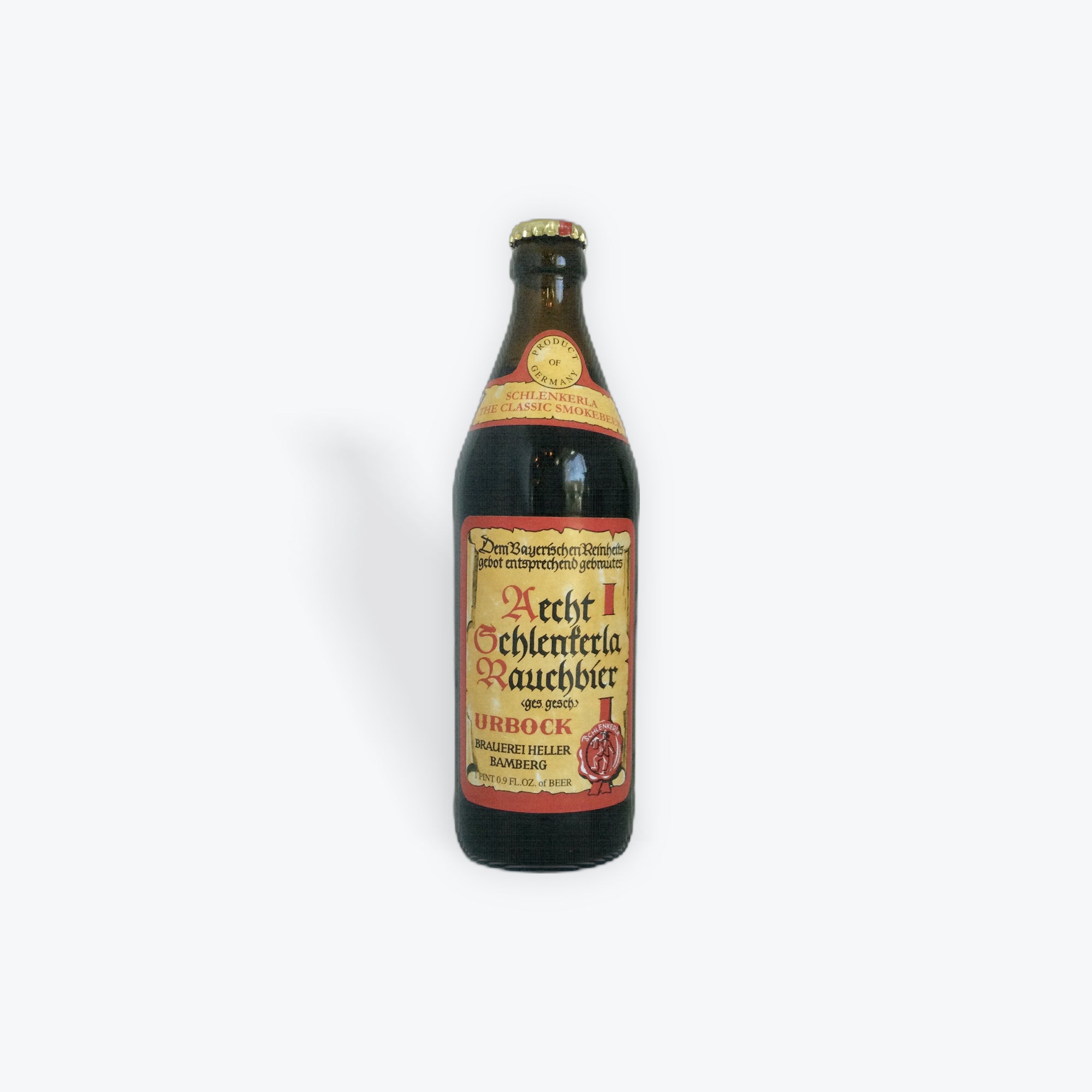Here we have a detailed close-up image of a dark brown glass beer bottle set against a white background. The bottle features a metal cap, indicative of one requiring a bottle opener. Dominating the forefront of the label is the word "Urbock" in red lettering, accompanied by "Heller Bamberg." The label's design integrates a predominantly yellow and red color scheme, reminiscent of antiquated parchment, adorned with black, gothic-style script typical of traditional German design. At the top of the label, it clearly states "Product of Germany," and additional text declares it as "Schlenkerla, the classic smoke beer." A round seal towards the bottom of the label depicts a dancing figure, possibly in Lederhosen, contributing to the traditional aesthetic of the bottle. The intricate details and classic German elements on the label emphasize the heritage and authenticity of this "smoke beer" from Bamberg, Germany.